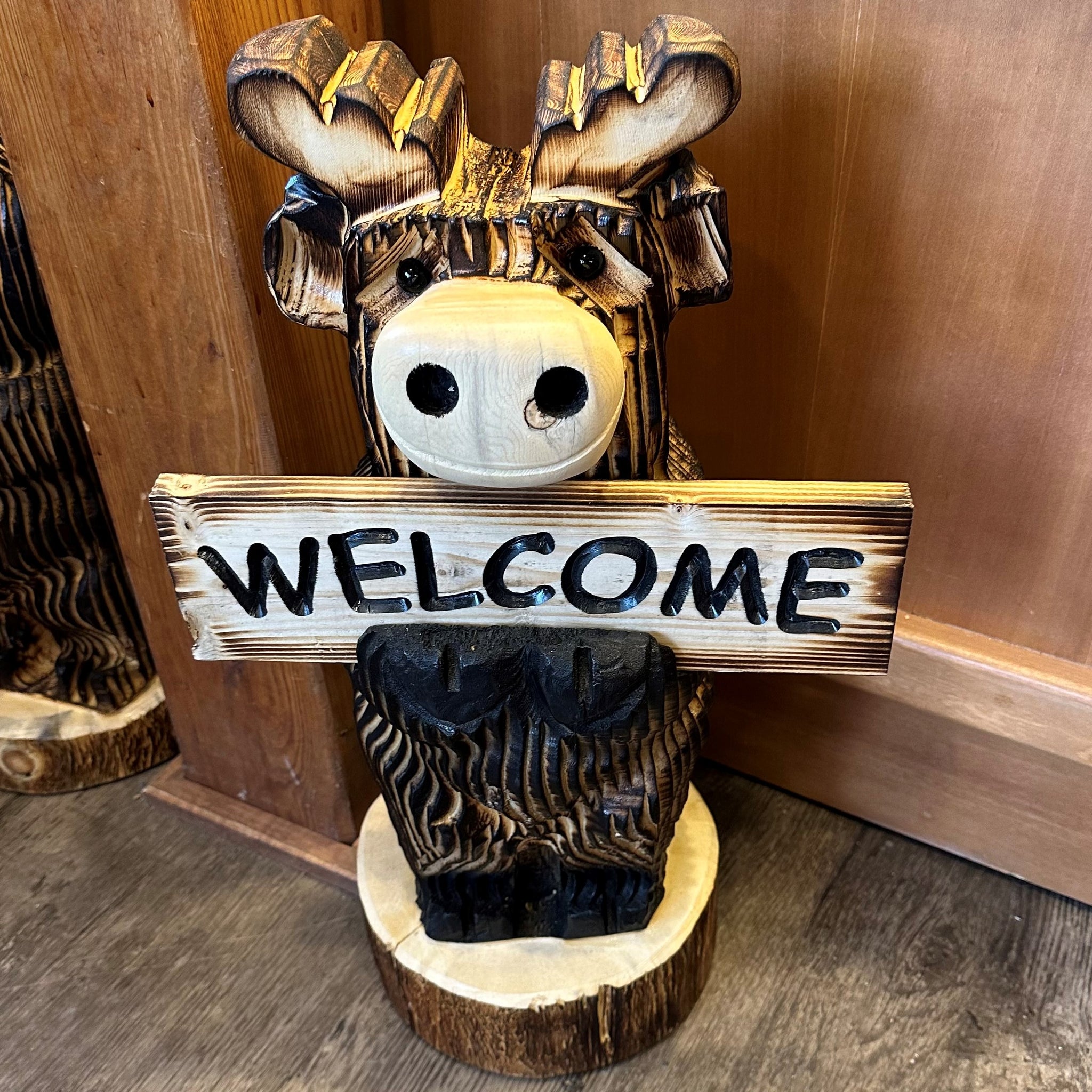This image showcases a detailed wooden carving of a reindeer, though sometimes mistaken for a moose. The reindeer is skillfully crafted, primarily using a chainsaw, with wood burning techniques applied to add depth and color variation. The reindeer squats on a round stump, displaying its distinctive features such as cute black eyes, a white muzzle, and wide antlers with hints of yellow. In its front hooves, it holds a welcome sign with black-painted letters. The carving is rich in earthy brown tones, reflective of tree bark. The photograph is set inside a rustic building with an old wooden floor and wood-paneled walls with molding. In the background, partially obscured behind a column, there's a hint of another statue. Overall, the scene suggests a warm, inviting atmosphere, possibly within a lodge.